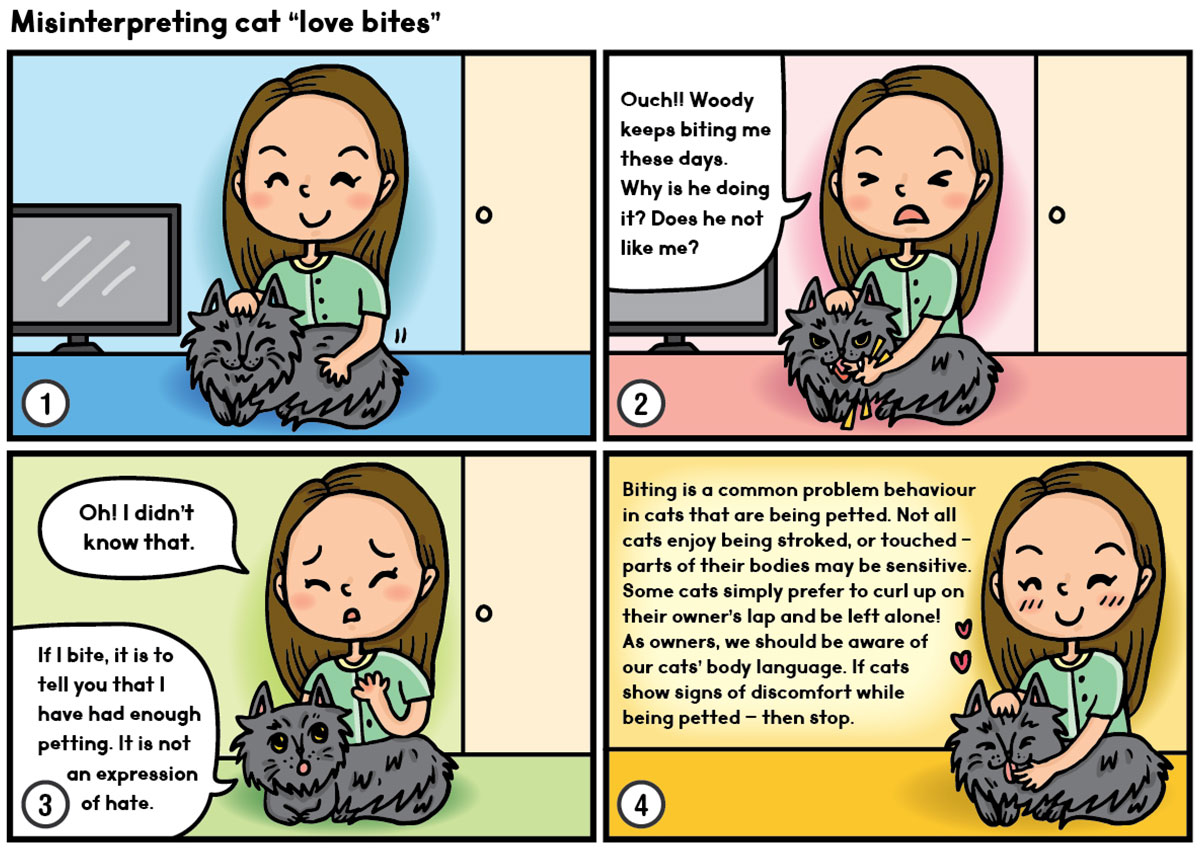This four-panel digital comic illustration, titled "Misinterpreting Cat Love Bites," educates on common feline behavior. The first panel, set in a blue-hued room, shows a girl with long brown hair and a green blouse petting a smiling gray cat, both appearing content. In the second panel, the scene changes to a pink background as the girl exclaims, "Ouch, Woody keeps biting me these days. Why is he doing it? Does he not like me?" In the third panel, tinged green, the cat explains, "If I bite, it is to tell you that I have had enough petting. It is not an expression of hate," to which the girl responds, "Oh, I didn't know that." The fourth panel features a yellow background with an educational note explaining that biting is a common behavior in cats being petted. Cats may have sensitive areas and may prefer to curl up on their owner's lap and be left alone. As owners, it is crucial to be aware of cats' body language and stop petting if signs of discomfort are shown. The comic concludes with the girl understanding and loving her cat, reinforcing the message about interpreting feline behavior correctly.